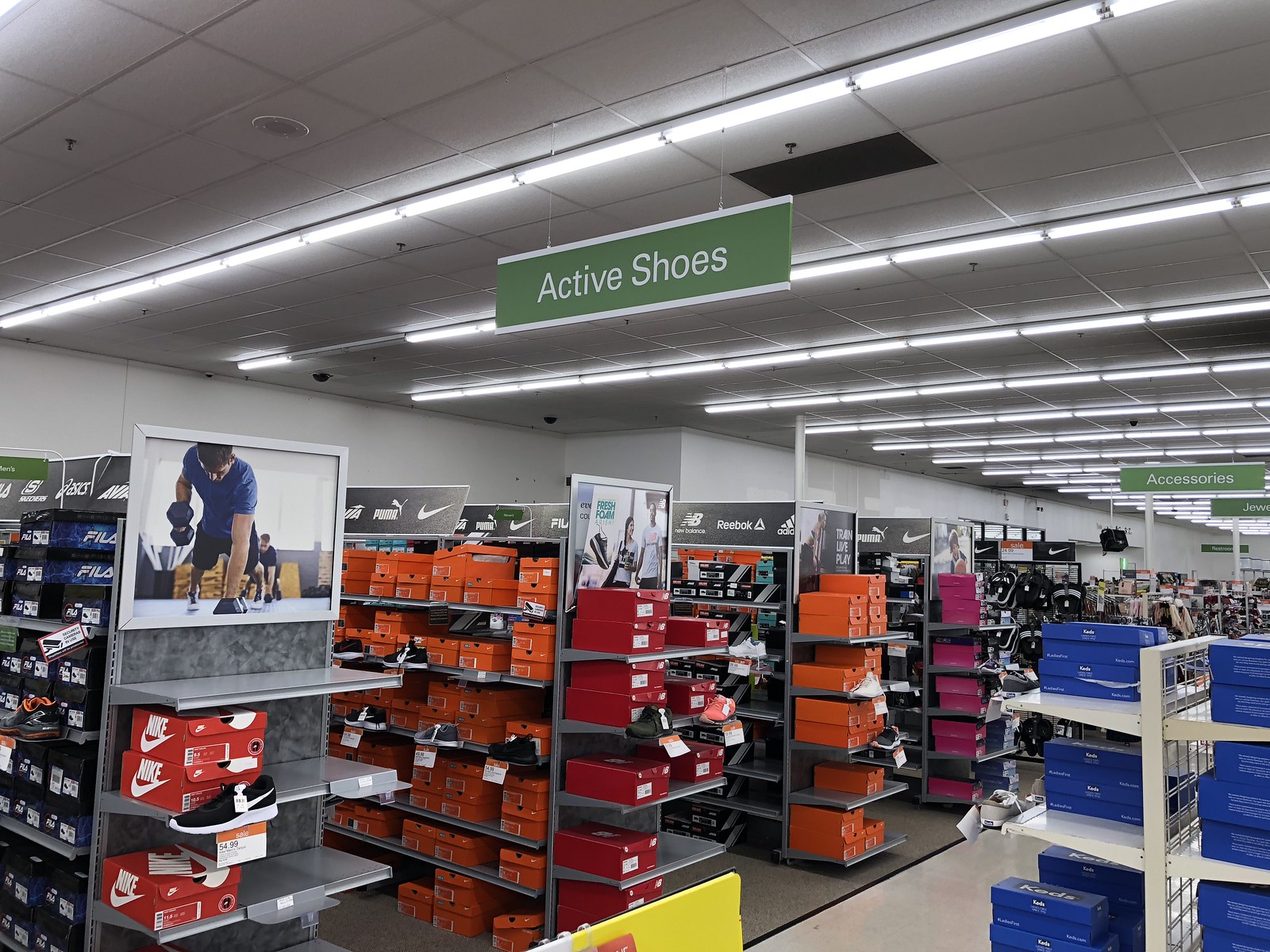This well-lit, horizontal photograph captures the interior of a shoe store, characterized by its commercial fluorescent lighting with bright, cylindrical light beams. The ceiling boasts white tiles, and prominently hanging from it are green rectangular signs indicating different sections. The most prominent sign, reading "Active Shoes" in white text, is followed by others further back, marked "Accessories" and "Jewelry."

On the left side of the store, multiple aisles are lined with shelves stacked with various shoe boxes. The nearest shelf features red cardboard boxes with the Nike logo. Adjacent shelves hold orange boxes, while subsequent ones display Reebok shoes in black and orange packaging. On the bottom right, there's a smaller white shelf displaying blue cardboard shoe boxes. The overall scene portrays a clean, well-organized store filled with a variety of shoe brands, including Nike, Reebok, and Puma, though notably devoid of any shoppers.